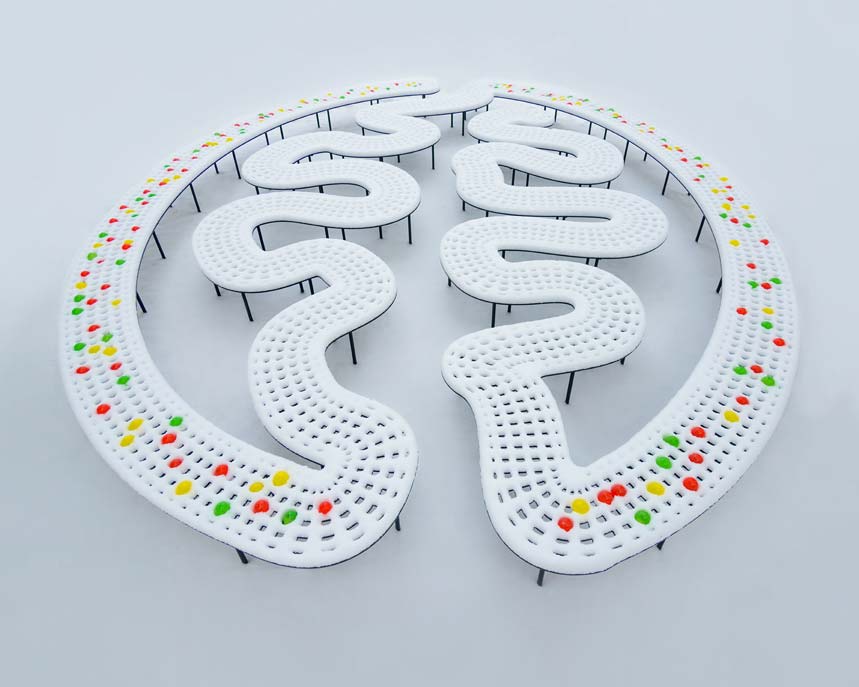The image depicts what appears to be a piece of modern art or an intricate, elongated bench that extends across a white background, possibly created by digital means. The structure has a somewhat elliptical shape overall, with a complex web-like or netted pattern made up of white material. Starting from half-circular sections on the left and right, the pattern rises and falls, forming snake-like zigzags until it converges in the center. The netting, gridded in texture, is detailed with multicolored dots—red, yellow, and green—strategically embedded along its outer loop but absent from the interior sections. Supporting this intricate network are numerous thin black legs extending underneath, giving it a delicate, almost floating appearance. The entire assembly could be interpreted as a combination of artistic and functional design, resembling a piece of furniture or a conveyor belt with slots that hold colorful elements.